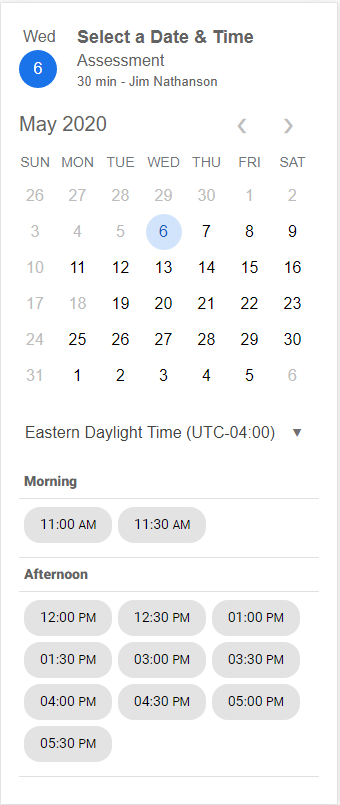A screenshot of a digital calendar interface from a device such as a laptop, smartphone, tablet, or desktop. At the top, there's a dark blue circle with a white number "6" inside it, representing the date. Above the circle, "WED" is displayed in gray text, indicating Wednesday. To the right, in black text, it prompts the user to "Select a date and time."

Below, it displays "Assessment" in bold black text, followed by "30 MIN" for the duration, and "Jim Nathanson" in regular black text. "May 2020" is shown as the month, with navigational arrows on either side to browse through different months. The top part of the calendar lists the days of the week: Sunday, Monday, Tuesday, Wednesday, Thursday, Friday, and Saturday. The calendar features all the days in May, with a light blue circle around the number "6" under Wednesday, marking the selected date.

At the bottom, it notes the time zone as "Eastern Daylight Time (UTC-04:00)" with a dropdown arrow beside it. Beneath this, "Morning" is highlighted in bold black, listing two available times in ovals: "11 a.m." and "11:30 a.m." Following this, an "Afternoon" section lists available times: "12 p.m.," "12:30 p.m.," "1 p.m.," "1:30 p.m.," "3 p.m.," "3:30 p.m.," "4 p.m.," "4:30 p.m.," "5 p.m.," and "5:30 p.m."